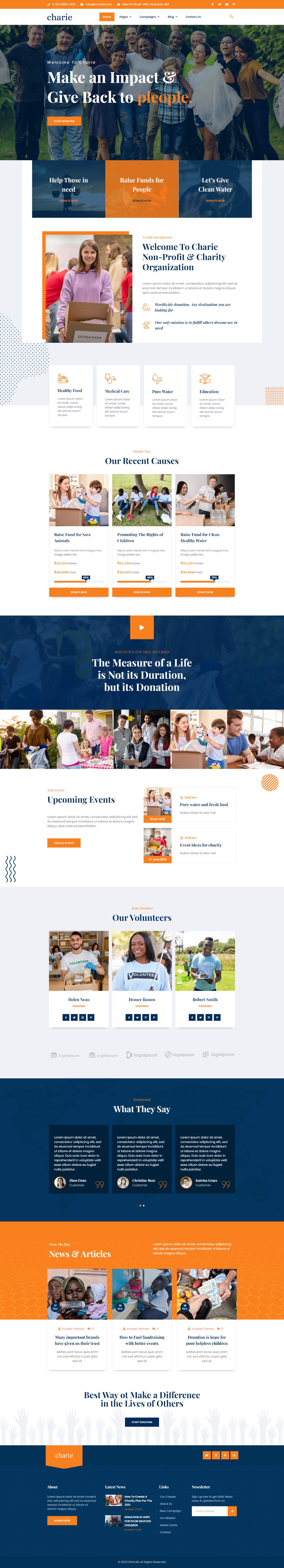The image comprises a vertically elongated, rectangular layout resembling a webpage's full-length screenshot. 

**Top Section:**
- An orange horizontal band crowns the top of the image.
- Immediately below, a muted color photograph features a group of people positioned horizontally.
- Beneath the photo, there are three sequential rectangular blocks: blue, orange, and blue, likely serving as selectable options or navigation elements.

**Upper Middle Section:**
- To the left, a picture of a woman donning a purple shirt is displayed.
- Below this image are four white rectangular areas filled with fine print.
- Extending horizontally in a row, three more images come next, each accompanied by fine print descriptors.

**Middle Section:**
- A dark blue border with white text serves as a section heading.
- Below the heading, several photographs are arranged horizontally, each featuring different individuals.

**Lower Middle Section:**
- A white area with touches of orange accents and fine print spread across fills the section.
- Beneath this, three pictures are aligned horizontally within a pale gray rectangle. The rightmost photo depicts a man in a blue shirt against a grassy and sky backdrop, the central image shows a woman in a light blue shirt, and the left picture features another person in a light shirt.

**Bottom Section:**
- Another horizontal dark blue band includes three squares with white fine print.
- Directly beneath, an orange band continues the horizontal alignment and includes three images.
- A substantial white area with fine print follows, leading to a concluding dark blue band at the bottom.
- This final band contains various selectable options marked by orange rectangles and fine print in white letters, accompanied by small images and a horizontal white bar that seems designed for data entry.